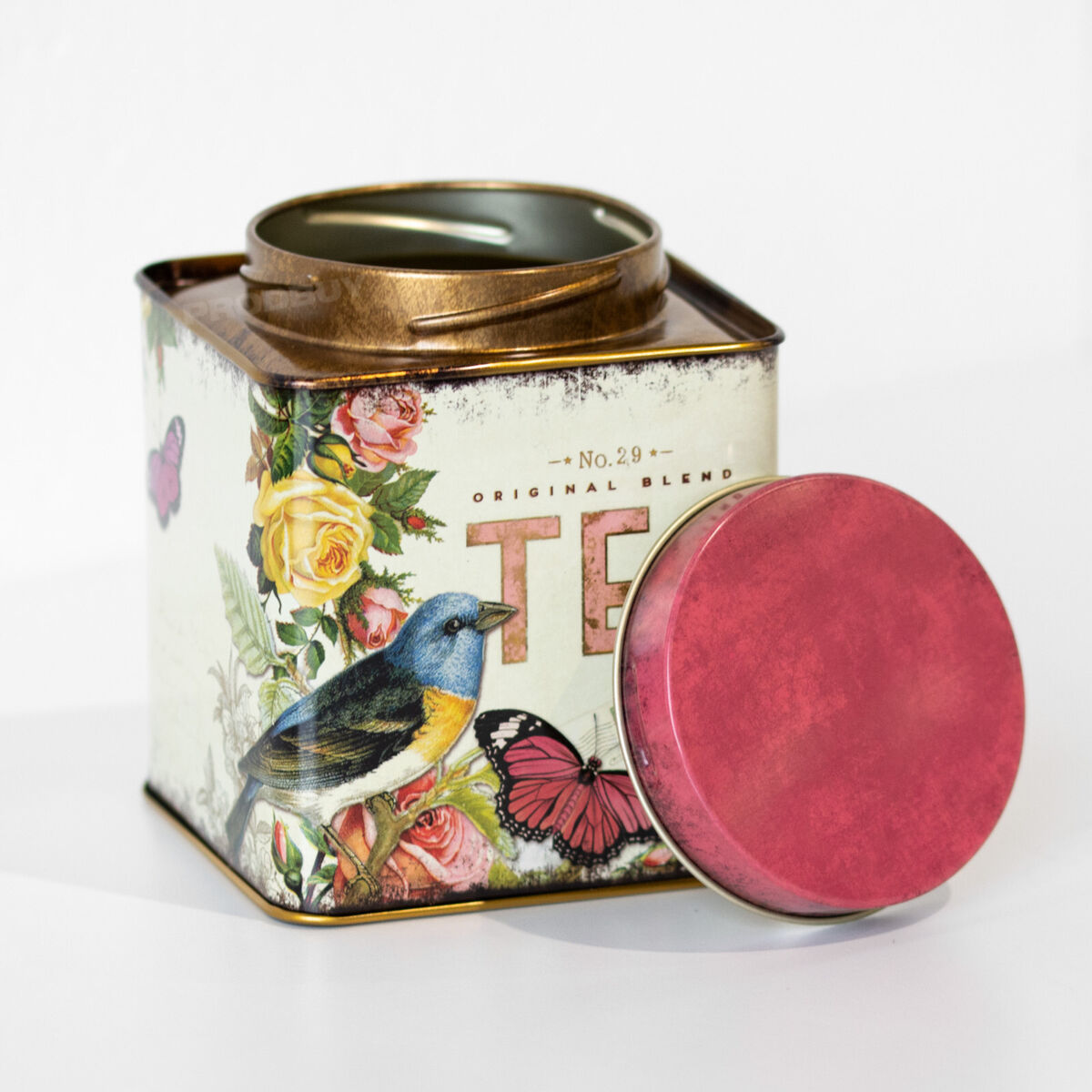The image depicts a large square picture with a solid light gray background, showcasing an old, cubical metal tea tin resting on a similarly colored light gray countertop. The face of the tin is adorned with intricate designs, featuring a bird with a blue head, dark gray or black feathers highlighted by a yellow under its neck, and a white belly. It is surrounded by pink and yellow flowers with green leaves and a butterfly located at the bottom center. Additionally, a purple butterfly is present on the left side of the tin. The tin is marked with the text "Number 29 Original Blend Tea," though the full word "Tea" is partially obscured because the pink screw-off lid is leaning against the container, revealing its dark brown, rusted metallic hue with a goldish tinge. Shadows from the lid fall onto the container, enhancing the vintage, worn appearance of the tin.